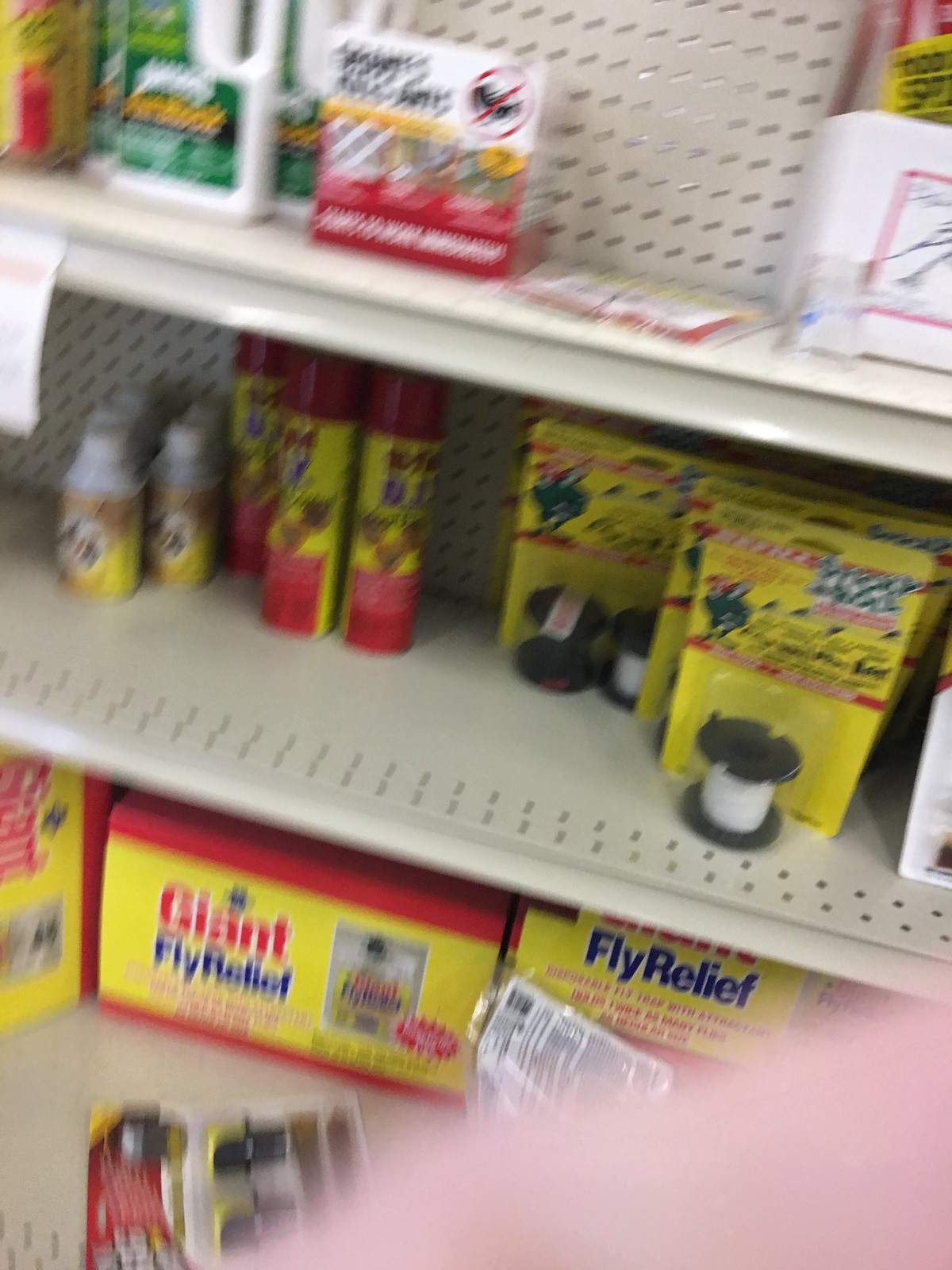The image appears to have been taken hastily inside what is likely a hardware store or a similar type of retail establishment. The photograph shows three shelves lined with various products, though the picture is somewhat blurry and includes a finger partially obscuring the bottom right corner, suggesting it may have been taken accidentally.

On the top shelf, there are canisters featuring red labeling that typically suggests hazardous or poisonous substances. One canister appears to sport a red symbol, possibly indicating its lethal nature or purpose. The middle shelf contains a product with packaging that includes an image of a mouse, hinting that it could be a rodenticide or mouse trap. The bottom shelf displays a product labeled "Giant Fly Relief," which is indicative of insect control solutions.

Overall, the shelves seem to be stocked with pest control products designed to address various household pests, including rodents and insects.